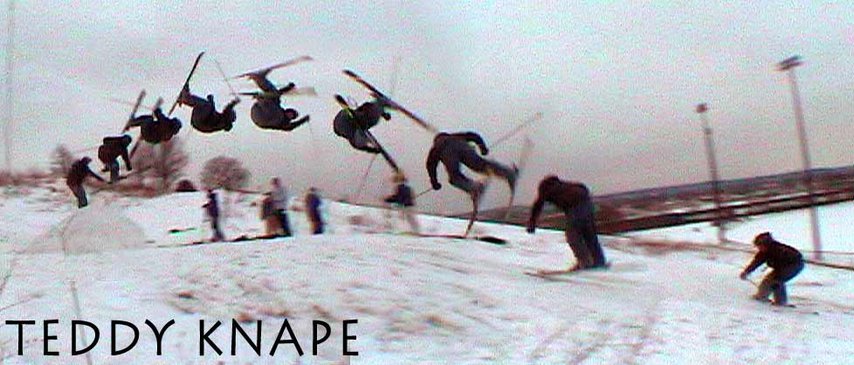A painting depicts a sequential motion of skiers performing a full flip. Positioned over a snowy bank with trees in the background, the scene vividly illustrates the progression of a skier's flip, starting from the far right where one skier is in the starting position, followed by another slightly lifted off the ground. The next skier is airborne, and the subsequent one is in mid-flip. The sequence continues with each skier showing a different stage of the flip until the final skier lands back on the ground. A family appears to be watching from the background, adding depth to the scene. The painting has a somewhat grainy texture, with slushy snow beneath the athletes. At the bottom left, in bold black capital letters, it reads "TEDDY KNAPP," emphasizing the artist's name.